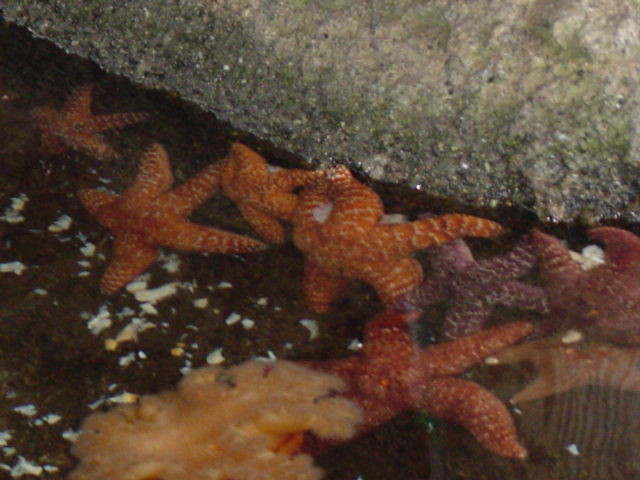The image captures a close-up view of eight starfish of various colors, such as vibrant oranges, deep browns, and reddish hues, clustered on and around a partially submerged, grayish-green rock with brown tinges. The rock, with its textured, rocky surface, appears to be underwater along an edge that rises above the waterline, creating little waves and splashes. The starfish, each with five arms, cling to the rock while immersed in the water, their hues contrasting against the stone. Specks and flecks are visible both on the water surface and beneath it, hinting at other underwater elements like potential seaweed. The scene, possibly photographed in an aquarium, highlights the serene interaction between the rock and the marine life.